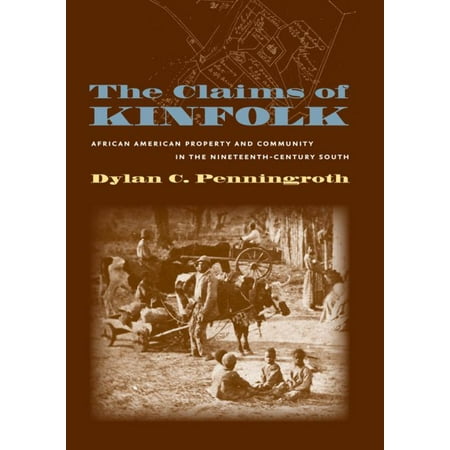Book cover description for "The Claims of Kinfolk: African-American Property and Community in the 19th Century South" by Dillon C. Pendergoth:

The cover has a brown background with a vintage effect. The title, "The Claims of Kinfolk," is prominently displayed at the top in blue font. Below the title, the subtitle "African-American Property and Community in the 19th Century South" is written in a smaller, centered white font, shifting alignment on each line. The author's name, Dillon C. Pendergoth, is also centered and appears just beneath the subtitle.

Covering more than half of the cover is an aged black-and-white photograph with a sepia tone that gives it a historical appearance. The image features a bustling farm scene set in the late 1800s, depicting various elements of African-American life during that period. African-American children are seen sitting in a circle on the ground, while men manage cows and oxen pulling carts. Women are engaged in different tasks around the farm. In the foreground, a man rides on a cart pulled by an oxen, and a woman stands next to a structure on the right-hand side. The scene also includes other farm details like a wagon wheel and utensils, capturing a moment that suggests both community and labor aspects of the past.